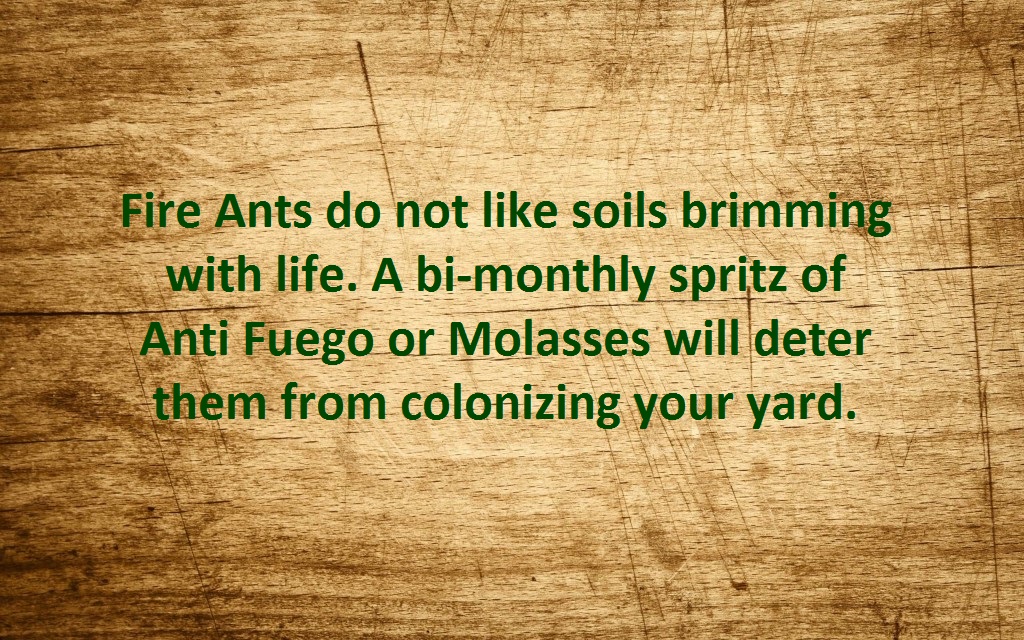The image is a promotional slide featuring a digital background that mimics a worn, cut-up wooden block or tabletop, characterized by various brown wood grains and numerous vertical cutting marks. At the center of this distressed wooden backdrop, there is an overlaid text in an army green color. The text consists of four lines, formatted in a bold, typewriter-like font. The message reads: "Fire ants do not like soils brimming with life. A bimonthly spritz of AntiFuego or molasses will deter them from colonizing your yard." This slide appears to offer a tip for preventing fire ants from invading one's yard.